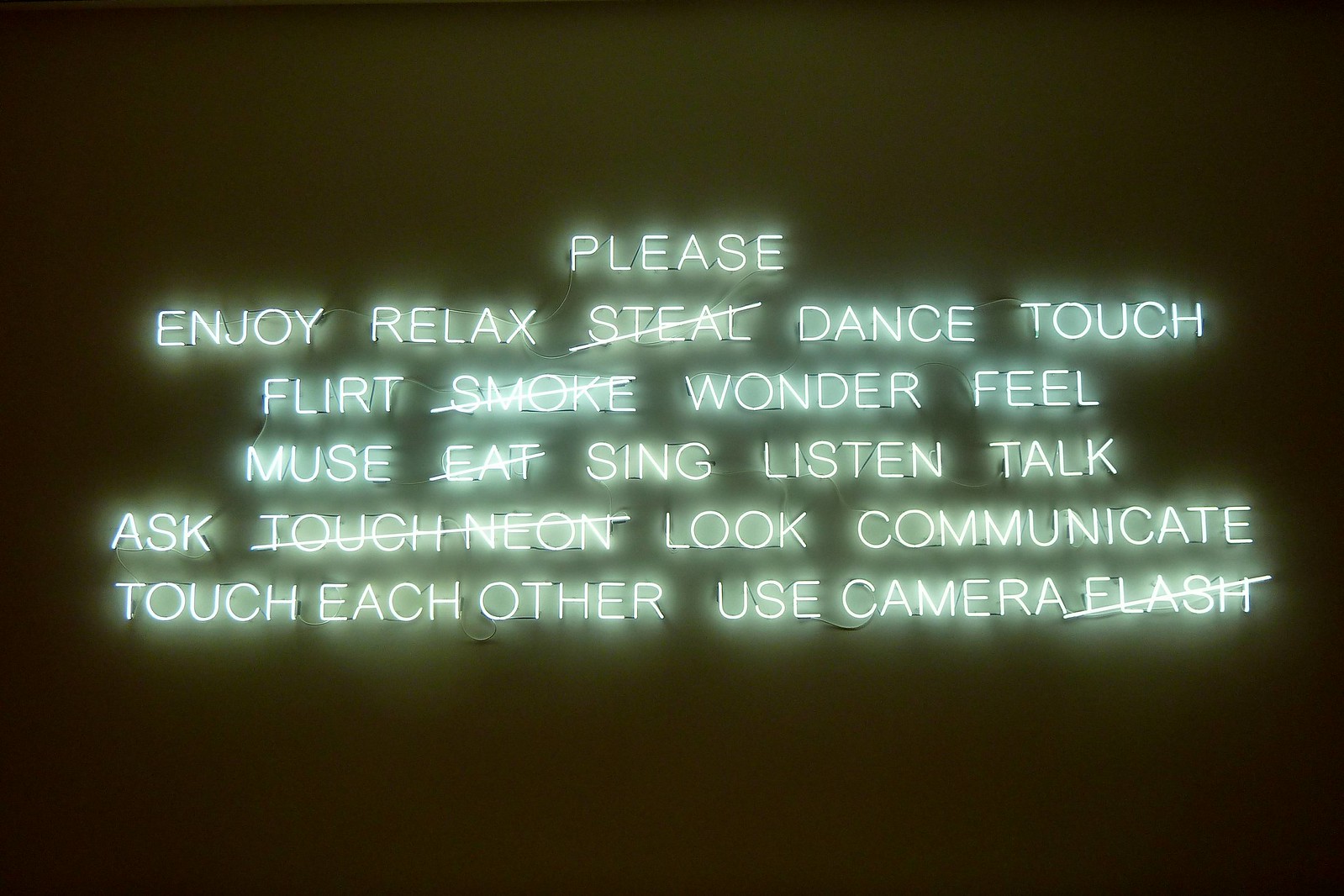This image presents a cleverly designed neon sign against a dark black background, potentially for a nightclub or bar setting. The sign features six lines of glowing green text with a white inner glow, resembling traditional neon lights. The text conveys a mix of actions to engage in and avoid, with the dismissed actions having a line through them.

The text reads:

Please
Enjoy, relax, ~steal~ , dance, touch
Flirt, ~smoke~ , wonder, feel
Muse, ~eat~ , sing, listen, talk
Ask, ~touch neon~ , look, communicate
Touch each other, ~use camera flash~ 

The graphic appears to be a set of playful and intriguing instructions, with a design that captures both a welcoming atmosphere and a sense of prohibition.